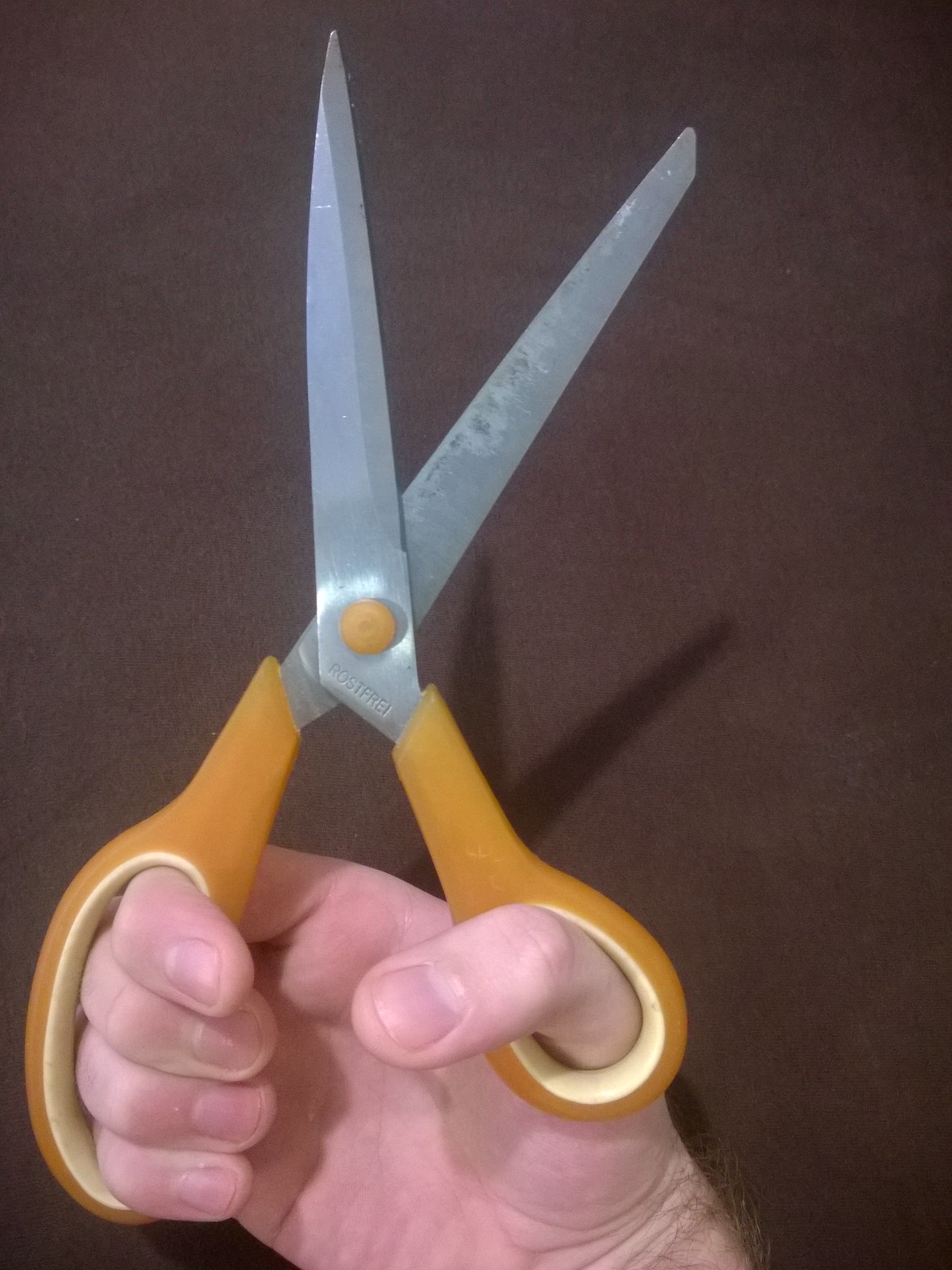In this image, we see a detailed close-up of a person's right hand holding a pair of large scissors. The hand is rotund with short fingernails and a light pinkish-white complexion, with brown hair visible on the wrist. The fingers are positioned through the orange and yellow handle holes of the scissors. The scissors themselves are made of silver steel with sharp, slightly dirty blades that cast a distinct shadow on a clean brown wall or rug in the background. The overall scene appears to be taken in a dimly lit room, suggesting the photo might have been taken in the afternoon or evening.